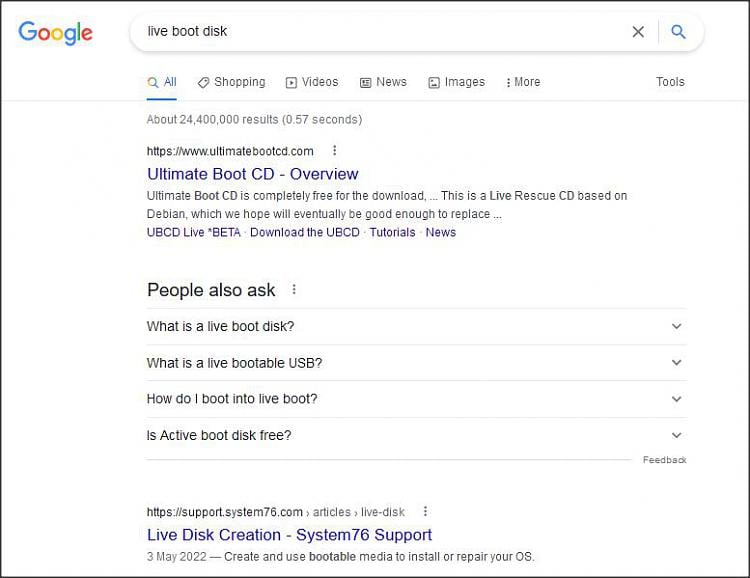The image depicts a screenshot of a Google search results page. It is a slightly rectangular shape, wider than it is tall. In the top left corner, the iconic Google logo is prominently displayed in its signature colors: blue, red, yellow, blue, green, and red. Below the logo is the search bar, containing the query "live boot disk."

Below the search bar, navigation options are listed: All, Shopping, Videos, News, Images, More, and Tools, with "All" being the highlighted selection. A gray line separates these options from the search results displayed further down.

Just beneath the navigation options, the results overview indicates approximately 24.4 million results found in 0.57 seconds. The first search result titled "Ultimate Boot CD Overview" provides a brief description and a link to the related website.

Directly below the first result, the "People also ask" section presents a list of frequently asked questions, including:
- What is the live boot disk?
- What is a live bootable USB?
- How do I boot into live boot?
- Is Active Boot Disk free?

Each question has a dropdown button on the right side, allowing users to expand and view additional information. Additionally, there is a small gray 'Feedback' button situated below these dropdowns.

The second search result listed is "Live Disk Creation - System76 Support," accompanied by a brief description and a link to the System76 support article.

The overall layout is typical of a Google search results page, effectively displaying relevant information and resources related to the search query "live boot disk."